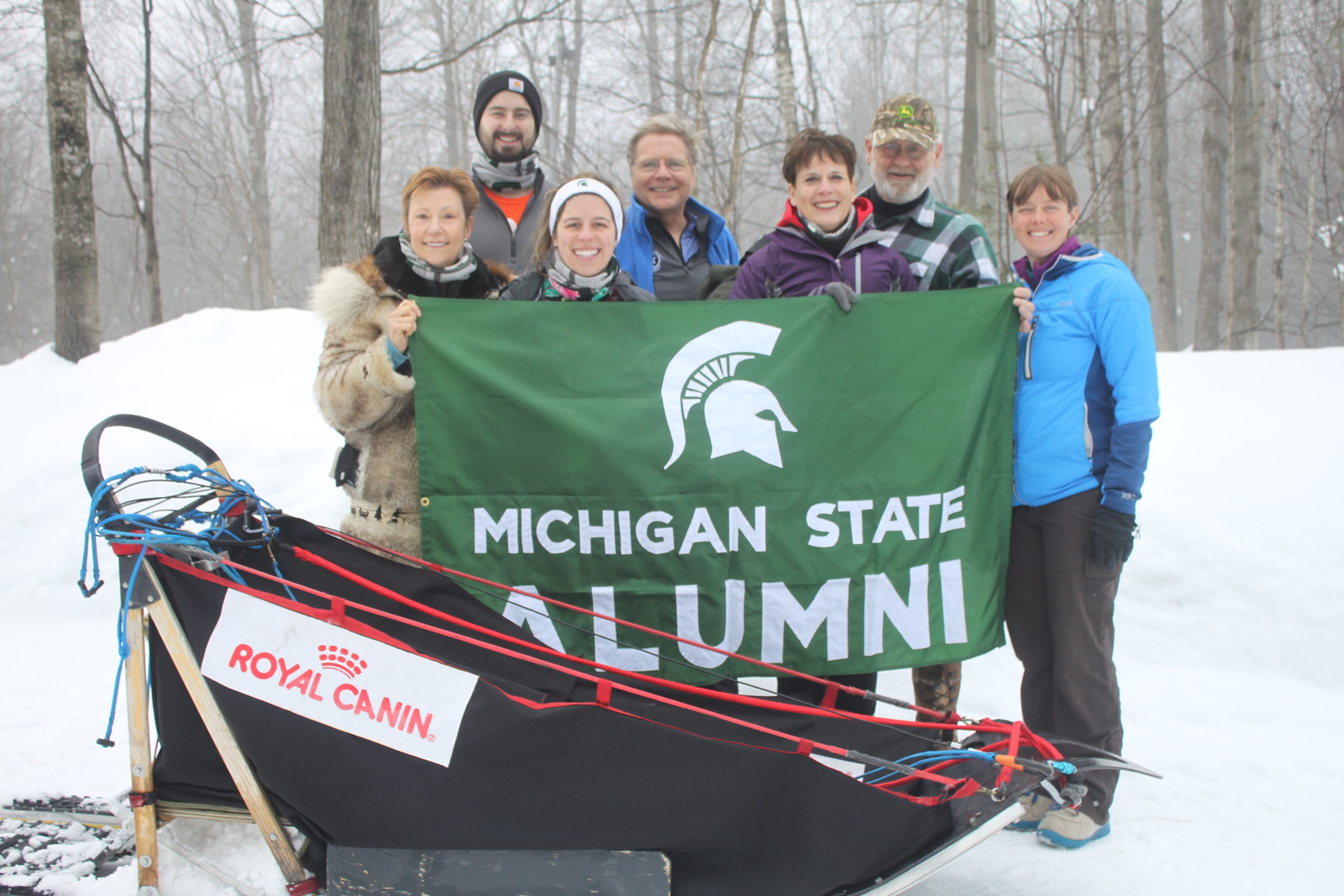In the photograph, seven individuals stand at the center, all smiling and gazing directly at the camera. The group is clad in various winter jackets that range in color from blue and purple to brown and gray, indicative of a cold, snowy setting. At the front, there are four women, and in the background, three men, all seemingly middle-aged, likely in their 30s or 40s. 

They proudly hold a dark green Michigan State flag, prominently displaying a white, two-dimensional silhouette of a Spartan headgear, with "Michigan State Alumni" written below, partially cropped at the “A” of “Alumni.” In the foreground lies a black sled with red accents, equipped with gear and straps, and marked with a sign reading "Royal Canin" in red letters on a white background.

Behind them, a wintry landscape unfolds with mounds of snow covering the ground and numerous barren trees dotting the background, their limbs stark and leafless against a gray, overcast sky mostly obscured by the trees. Specific details of their attire include a lady on the right in a blue coat and black pants, a man beside her in a black, green, and white checkered shirt with a John Deere cap, a woman in a purple jacket, another man in a blue coat and black shirt, a lady with a white headband and black coat, a gentleman in a gray jacket with an orange shirt and black beanie, and finally, a lady in a brown winter coat on the far left. This image captures what appears to be a group of Michigan State alumni, gathered amidst a serene winter landscape, unified by their shared alma mater.